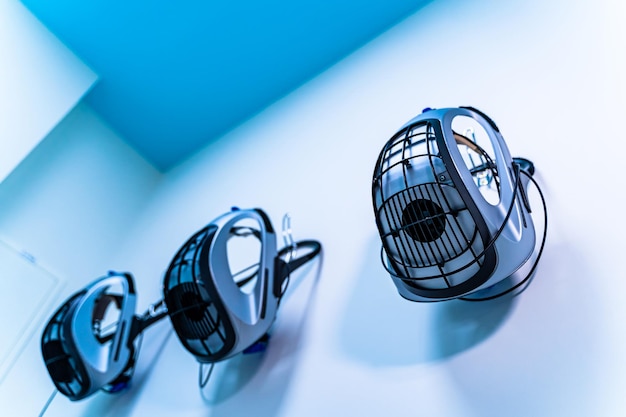The photograph presents a stylized, photorealistic image viewed from a skewed, upward-looking perspective. You can see a corner where two white walls meet, along with a light blue ceiling, all casting gray-blue shadows. The focus is on three identical, futuristic items hanging on silver hooks along the slanted wall. These objects have black, webbed grills over a shiny, possibly metal framework, each equipped with handles. While it's challenging to determine their exact purpose, they could be fans, blowers, or some form of protective gear due to their modern, sleek design. The image is devoid of people and primarily features shades of blue, black, and white, giving it a sci-fi aesthetic. The rightmost object is in sharp focus, while the two to its left gradually blur with distance.